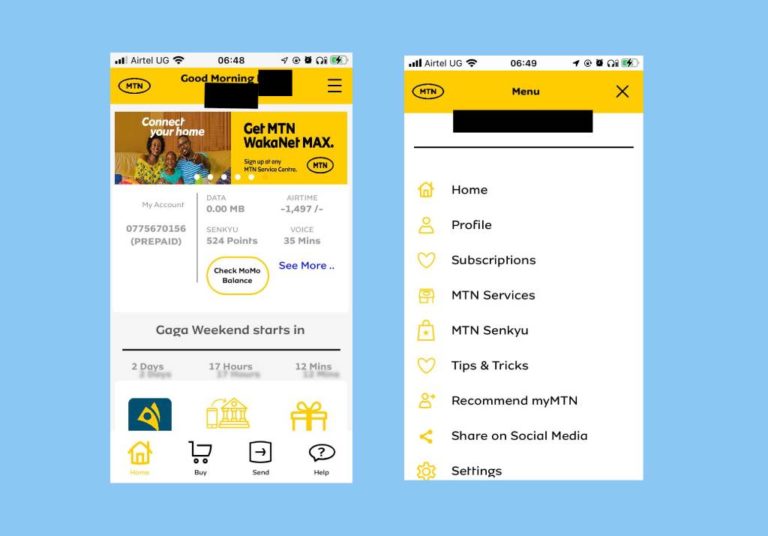The image captures the display of an iPhone showing various details on the screen. The battery life of the iPhone is approximately 50%, and it has a strong network connection provided by Airtel UG. The screen displays a greeting "Good Morning," next to which is a text box with the MTN logo in yellow. 

At the top of the screen, a banner reads "Connect Your Home" with an image of a Black family sitting together on a couch, promoting MTN Wakanet Max. The banner includes a call to action for signing up at any MTN service center or bank center.

Below the banner is account information indicating it is a prepaid account. The data usage is listed as zero, while the airtime balance is shown as negative 1497. The user has accumulated 824 points and has 35 minutes of voice call time remaining. There's a yellow circle marked "Check Momo Balance." An option to see more details is highlighted in purple.

Further down, a countdown timer indicates that a "Gaggle Weekend" starts in 2 days, 17 hours, and 12 minutes, accompanied by various small icon images including a present, a house, and what appears to be a fish. The bottom of the screen has navigation buttons for "Home," "Buy," "Send," and "Help."

The subsequent page includes sections labeled "Home," "Profile," "Subscriptions," "MTN Services," "MTN Thank You," "Tips and Tricks," "Recommended by MTN," "Share on Social Media," and "Settings."